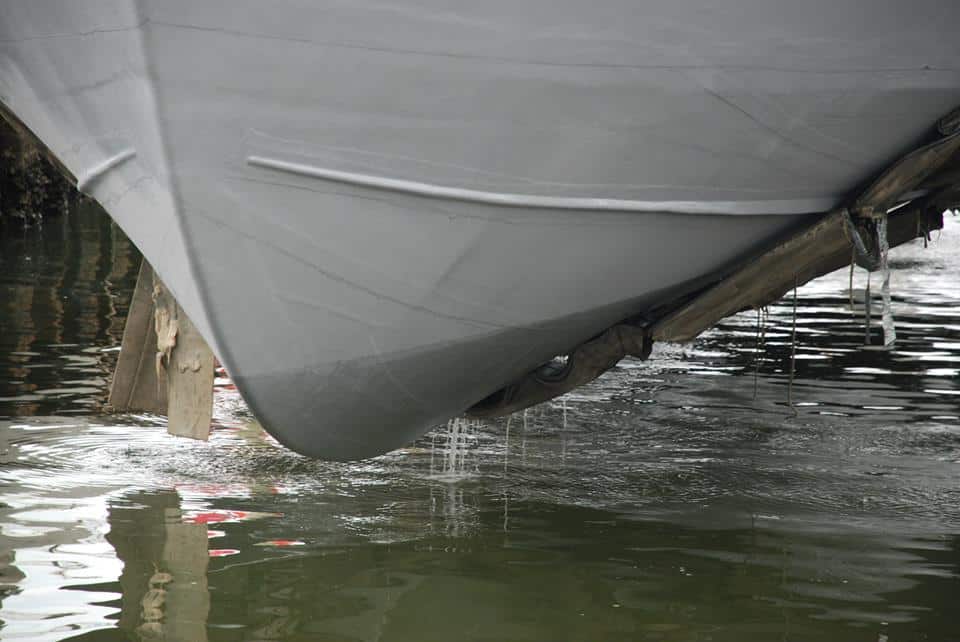The image captures the underside of a white boat prominently filling the frame from the top to the middle, appearing freshly hoisted out of the water. Water is visibly dripping or leaking from the hull back into the dark, gray-green body of water below, which reflects hues of white and red. A darker section is noticeable at the bottom of the hull, and a lifting mechanism is discernible, indicating the boat's recent elevation. On the left side of the photograph, part of a typical white wooden dock and its reflection are visible, further grounding the scene in a marina-like setting.